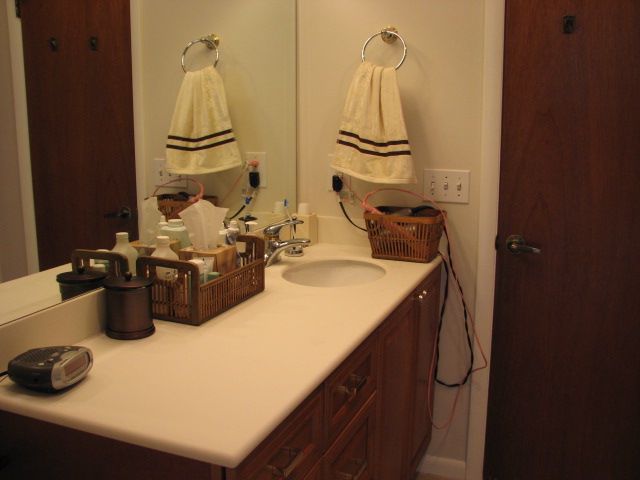This photograph captures a cozy bathroom bathed in a warm orange glow, suggesting the presence of one or two lights casting a soft hue across the space. To the right, there's a brown door with a dark brown knob, above which hangs a towel hanger of a matching dark brown color. 

To the left of the door, a set of three light switches is visible, albeit from a distance; notably, the two switches on the right are flipped up, while the one on the far left is flipped down. Beneath these switches sits a basket with a pink handle, its exterior adorned with a wooden, stick-like design. Draped over the basket is a somewhat dirty, brownish-white rag marked by two blue horizontal lines near its bottom.

Moving leftward along the counter, which is immaculately clean, an alarm clock is positioned at the far end. Although the time isn't visible due to the angle, the clock itself features a black back and a gray front. The counter, along with the sink, is a pristine white, creating a striking contrast to the silver faucet knobs.